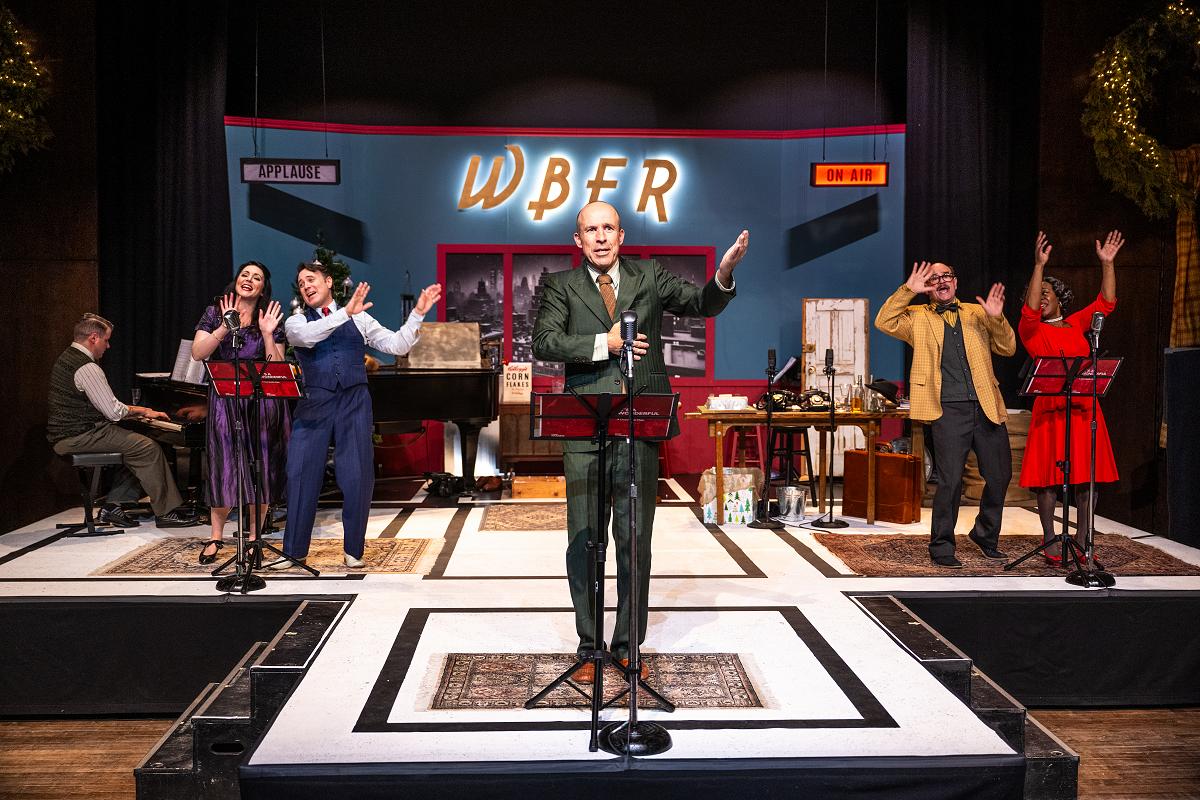The image, appearing almost like an AI-generated drawing due to its vivid colors, depicts a lively stage setting with a backdrop indicating a radio or TV station labeled "WBFR." Central to the scene is a bald man dressed in a suit and tie, standing at a microphone with one hand extended outward and the other on his chest, possibly addressing an audience beyond the frame. Flanking him are two pairs of performers, each behind a microphone and music stand; on the right is a woman with black hair in a red dress alongside a bald man in a gold jacket and black pants, both raising their hands as if singing. On the left, another pair of women is enthusiastically waving their hands. Behind them, a man in a vest and light shirt is seated at a piano on the far left, playing. The background is adorned with illuminated signs reading "APPLAUSE" and "ON AIR," suggesting a live broadcast, and adding to the theatrical ambiance. A table with a briefcase beneath it and various stage lights further complete the vibrant setting of this orchestrated performance.